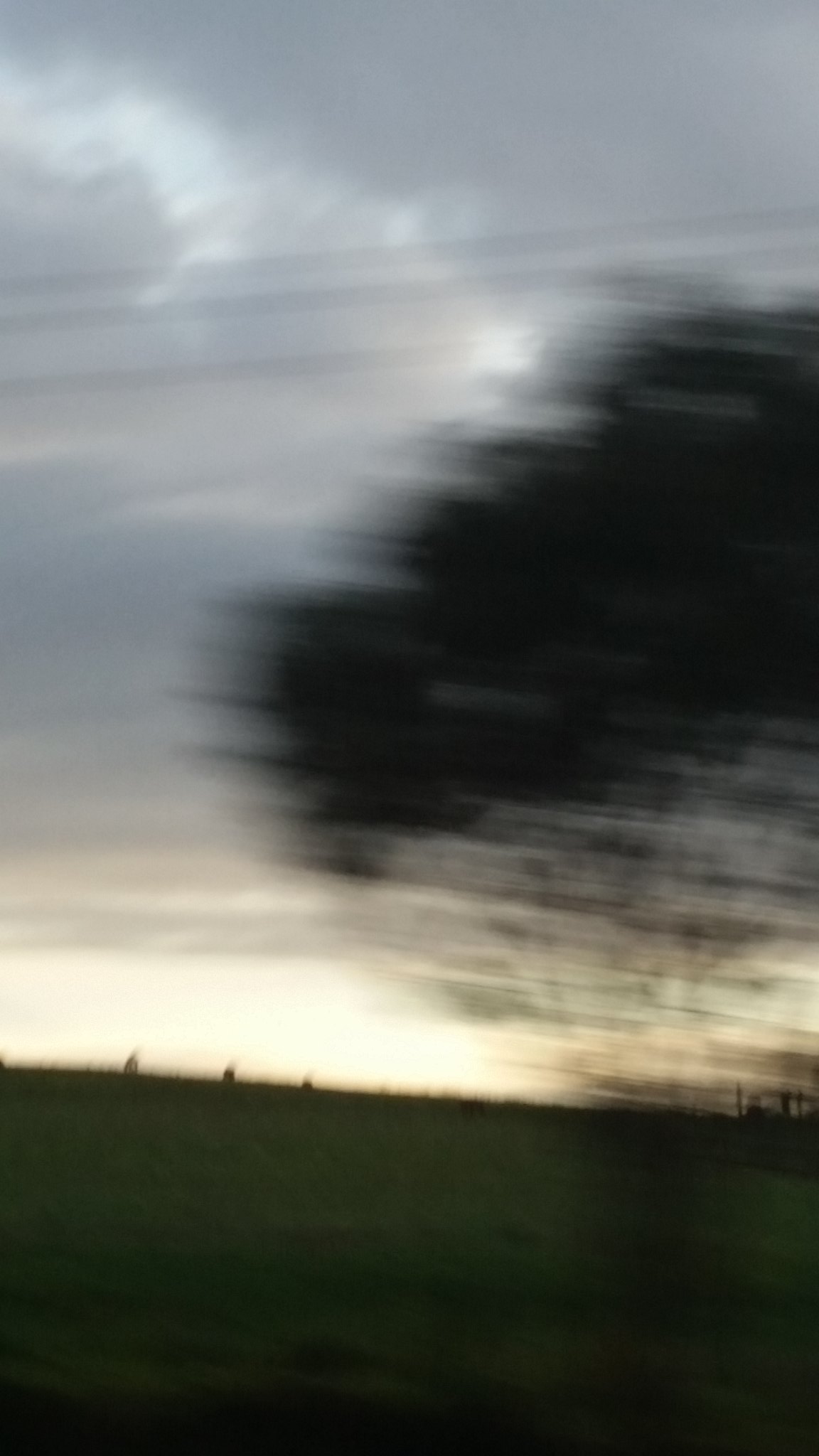The image features a predominantly gray sky with a contrasting white cloud cover at the top. On the right side, dark, intricately branched trees with black leaves create a stark silhouette against the lighter background. The center of the image is illuminated by a bright white light that gradually diminishes toward the edges. Power lines stretch horizontally across the upper segment of the frame, contributing to the composition's layered aesthetic. The bottom part of the image transitions into darker tones, with shadows and black areas creating a strong visual contrast with the lighter sections above.